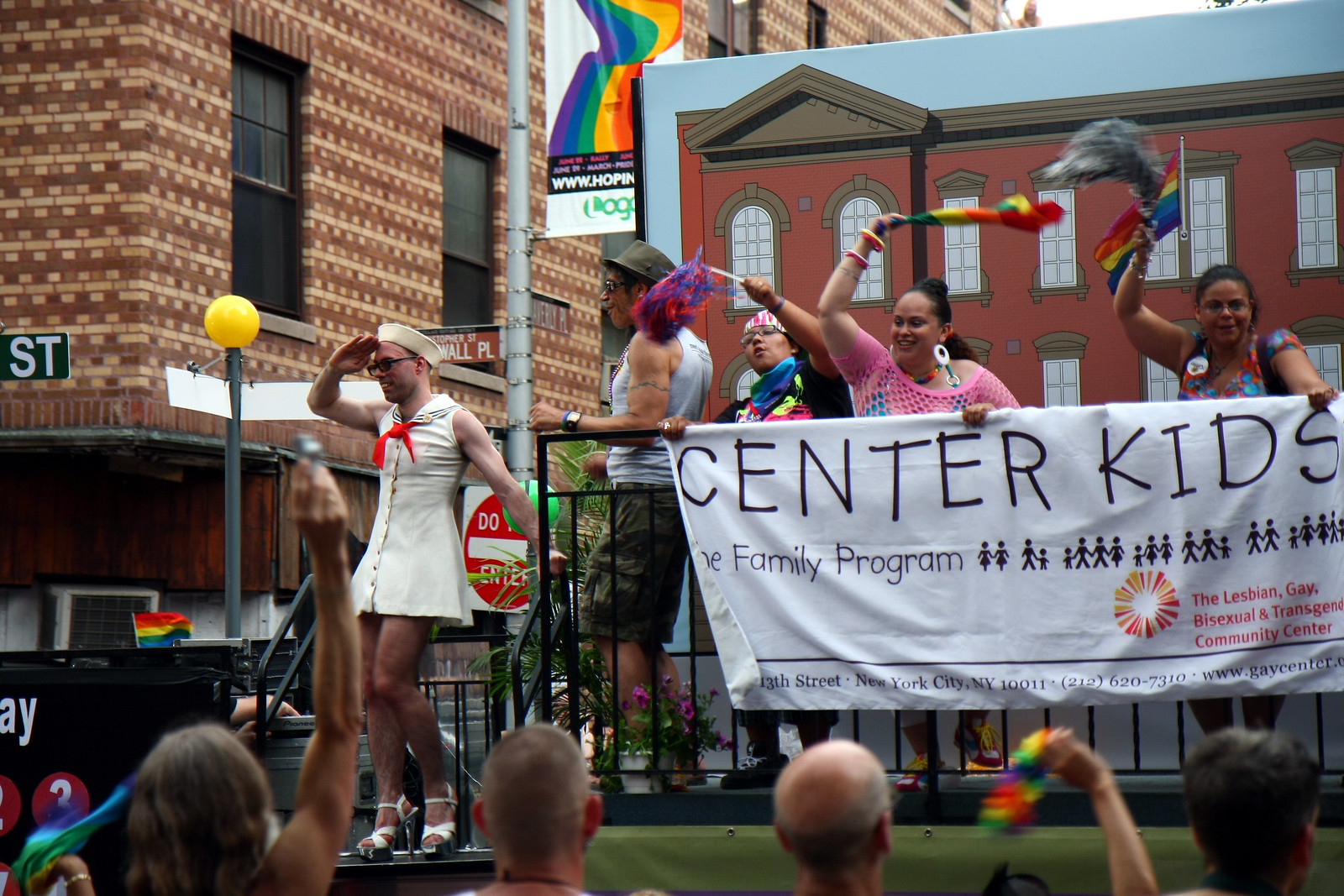The photograph captures a vibrant and lively scene from a gay pride festival, held outdoors in the middle of the day. Directly in the center of the image, a parade float takes prominence, resembling a house and adorned with a colorful banner that reads "Center Kids Family Program." The banner further promotes the cause by stating it is part of the Lesbian, Gay, Bisexual, and Transgender Community Center, and includes an address, a phone number, and a website. In the foreground, three jubilant women are seen holding the banner, clearly in enthusiastic support of the cause. To the left of the float, a gentleman dressed in a distinctive outfit consisting of a dress and a navy hat adds to the festive atmosphere. The background features several buildings, likely including the community center itself, and a street sign, all under a clear, warm sky. The scene is filled with individuals, many clad in rainbow-colored attire, symbolizing their solidarity with the LGBTQ+ community. The crowd's energy is palpable, with people in the foreground cheering, raising their arms, and embodying the spirit of celebration and support for the cause.